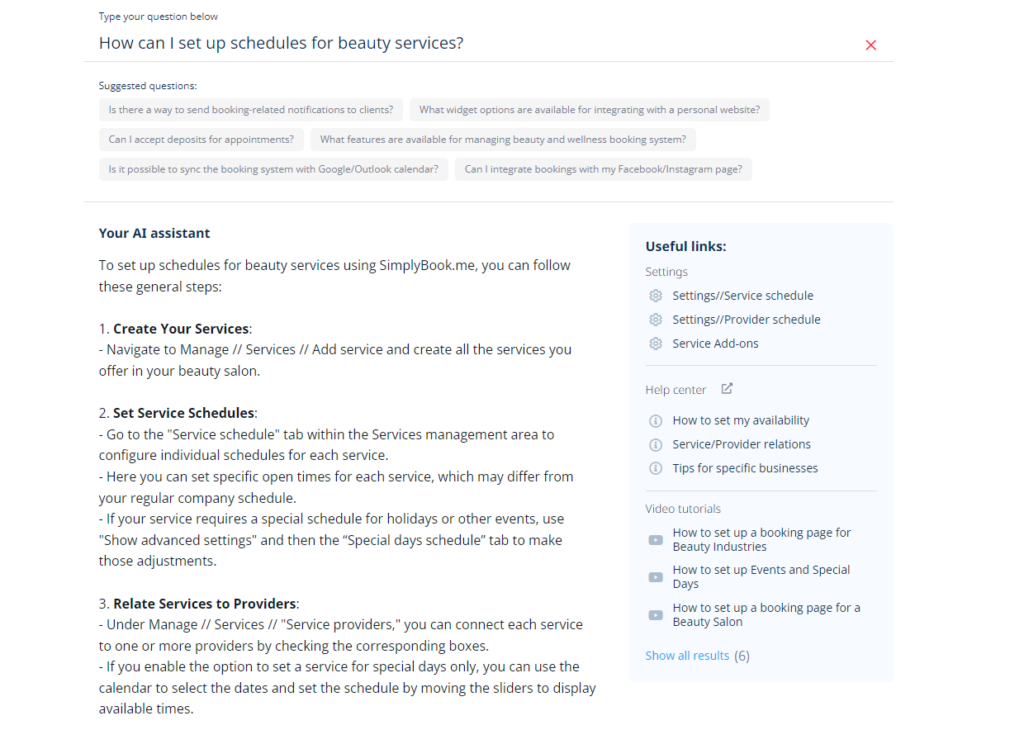The image depicts a user interface displaying a search query about setting up schedules for beauty services. At the top, a small text prompt invites users to "type your question below." The user has queried, "How can I set up schedules for beauty services?" followed by a question mark. A horizontal line acts as a separator below the query. 

Underneath the line, there are suggestions for related questions that the user can explore. Further down, the interface provides a detailed response from an AI assistant on how to set up schedules for beauty services. The response outlines three main steps:

1. **Create Your Services**: Navigate to the 'Manage Service' section, then add and create all the services your beauty salon offers.
2. **Set a Schedule**: Define the scheduling parameters for your services.
3. **Relate Services to Provider**: Link the services to the respective providers.

On the right side of the image, there are several useful links that provide additional information and resources related to the initial question, offering further assistance to the user.